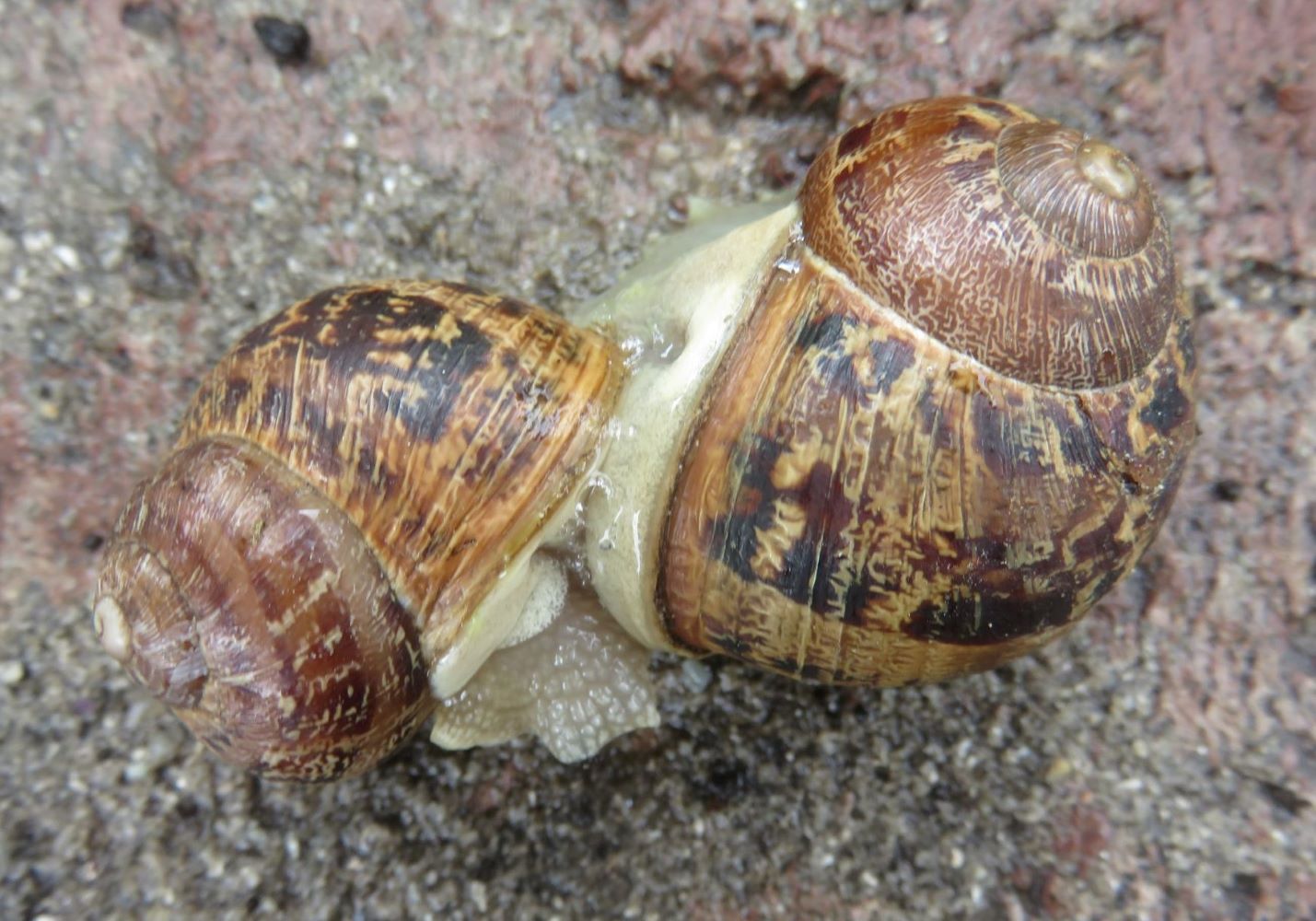In this close-up photograph taken outdoors, we see two snail shells that are closely positioned, possibly indicative of mating or interaction. One shell is noticeably larger than the other, and they are connected by a sticky, yellowish goo with a white, slightly scaly-looking mass visible between them, likely part of the snail. The shells themselves are predominantly brown with varied streaks of lighter brown and black, featuring a spiral pattern. They rest on a surface composed of reddish-brown gravel and sand, with darker sediments scattered around, in a setting illuminated by natural but indirect light. The detailed texture of the ground and the intricate patterns on the shells create a vivid, detailed scene that highlights the natural elements and interactions of snail life.